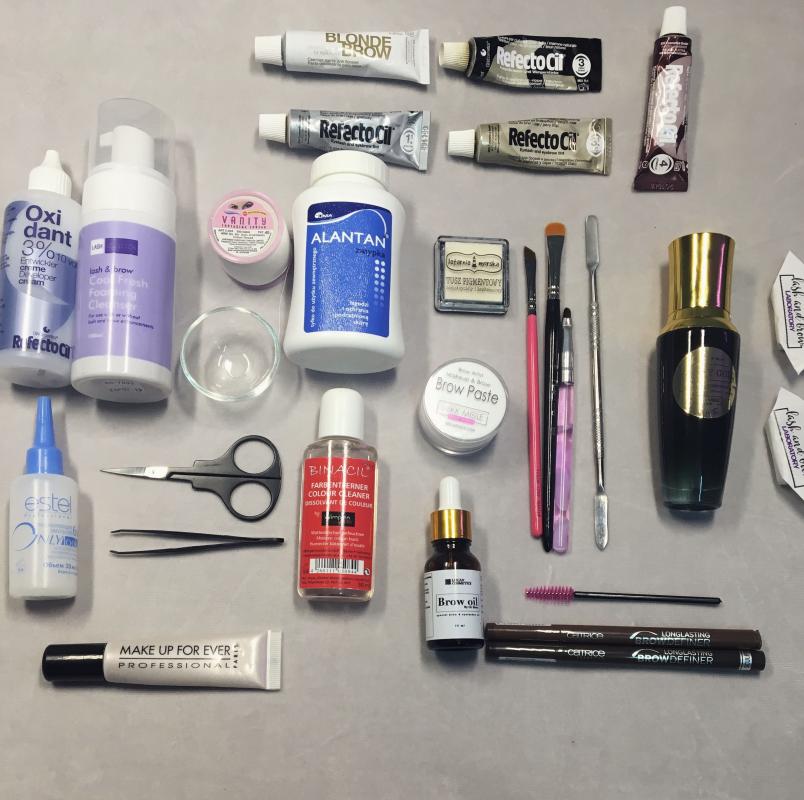The image meticulously showcases an array of health and beauty items artfully arranged on a light gray countertop. At the top, four tubes resembling toothpaste are neatly placed in two rows of two. The top left tube, white and labeled "Blonde Brow," stands out among three tubes of "RefectoCil" products in varying shades—silver on the lower left, bronze on the lower right, and a bronzed-black mix on the upper row. These tubes are each marked with numbers 1 through 3. Completing this group, a fourth "RefectoCil" tube labeled 4 is positioned vertically in the upper right corner.

Beneath this, a striking black bottle with a gold cap catches the eye, flanked on the left by an assortment of brushes and nail tools. Adjacent to these is a cylindrical container of brow paste accompanied by a white square with faint writing. Shifting further left, a blue bottle marked "Alantan" sits beside a cylindrical container labeled "Vanity," a small empty bowl, and a pump-topped container in white and purple that reads "Cool Fresh Foaming Cleanser." Continuing the arrangement, a "RefectoCil" bottle labeled "Oxidant 3%" is followed by a blue and white bottle from "Estel" placed on the image's left edge.

Just next to the Estel bottle, a pair of precision tweezers and a small pair of scissors rest neatly. Below lies a tube from "Make Up For Ever Professional" with a black cap. To the right of the scissors and tweezers, a bottle labeled "Benicil" with a red label is prominently displayed alongside a dropper-topped bottle designated "Brow Oil."

Rounding out the lower right section, a spoolie brush is positioned next to two slim, cylindrical containers of eye products, completing the well-organized and comprehensive selection of health and beauty items.